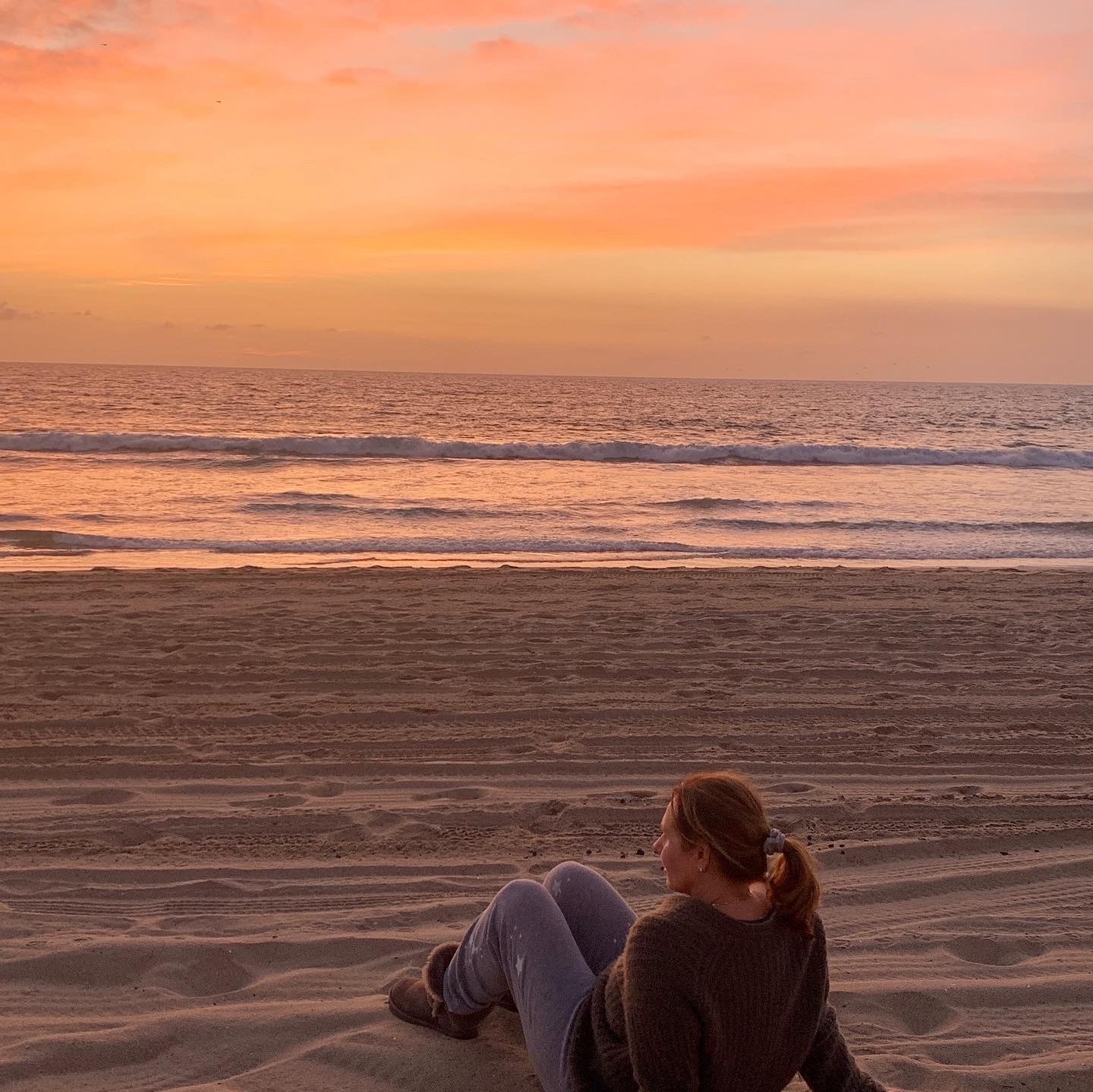In this picturesque scene, a fair-skinned woman in her 20s sits peacefully on a sandy beach, facing the horizon where the sky displays a mesmerizing sunset of pastel pinks, oranges, yellows, and soft beiges interspersed with wispy clouds and faint patches of blue. Her blonde hair is pulled back into a ponytail with a light brown scrunchie, and she is dressed warmly in a knitted dark brown long-sleeve sweater, blue jeans, and brown ankle-height winter boots that look like UGGs. She sits comfortably, leaning back on the sand, possibly indicating it is either a chilly spring evening or early morning. The gentle waves break about 40 to 50 feet from shore, enhancing the serene atmosphere with their calm rhythm. The beach, mostly undisturbed except for various track marks, is as tranquil as the moment she seems to be deeply absorbed in, giving the impression of solitude and contemplation.